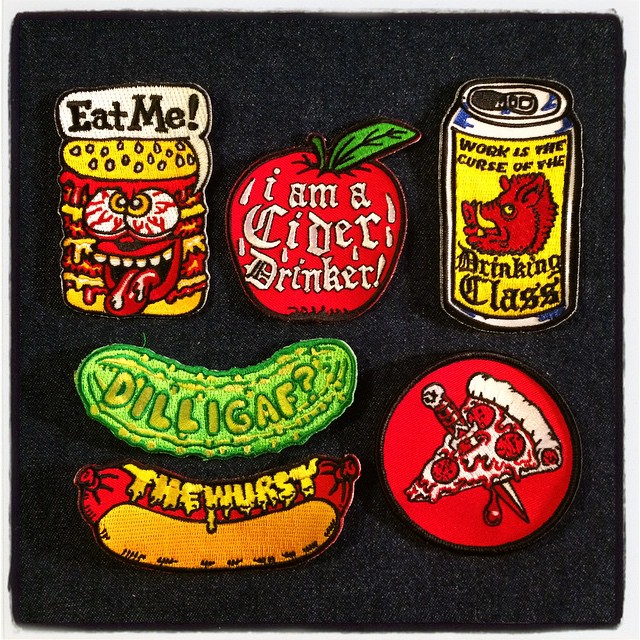The image depicts a collection of six vibrant and quirky iron-on or sew-on patches displayed on a gray carpet background. The first patch on the top left showcases a whimsical hamburger with a maniacal expression, featuring googly eyes, a Rolling Stones-style tongue, five teeth, bloodshot eyes with yellow pupils, and the phrase "Eat Me!" in bold black letters on a white background. Below it is a red apple with a green stem, inscribed with "I am a cider drinker" in white letters.

Next, there is an aluminum beer can with a label featuring a snarling boar's head, complete with yellow tusks and eyes. The boar’s red fur is accented with black trim, and the can bears the phrase "Work is the curse of the drinking class." The fourth patch is a playful green pickle with the words "DILLYGAFF" (a humorous acronym for "Do I Look Like I Give A F***") in black letters.

Following the pickle is a hot dog nestled in a golden bun, complemented by the phrase "the wurst" written in a mustard-like font above it. The final patch features a knife piercing through a slice of pepperoni pizza, bleeding tomato paste. The details and eclectic designs give off a raw, energetic, and fun-loving vibe, embodying a creative and whimsical spirit.